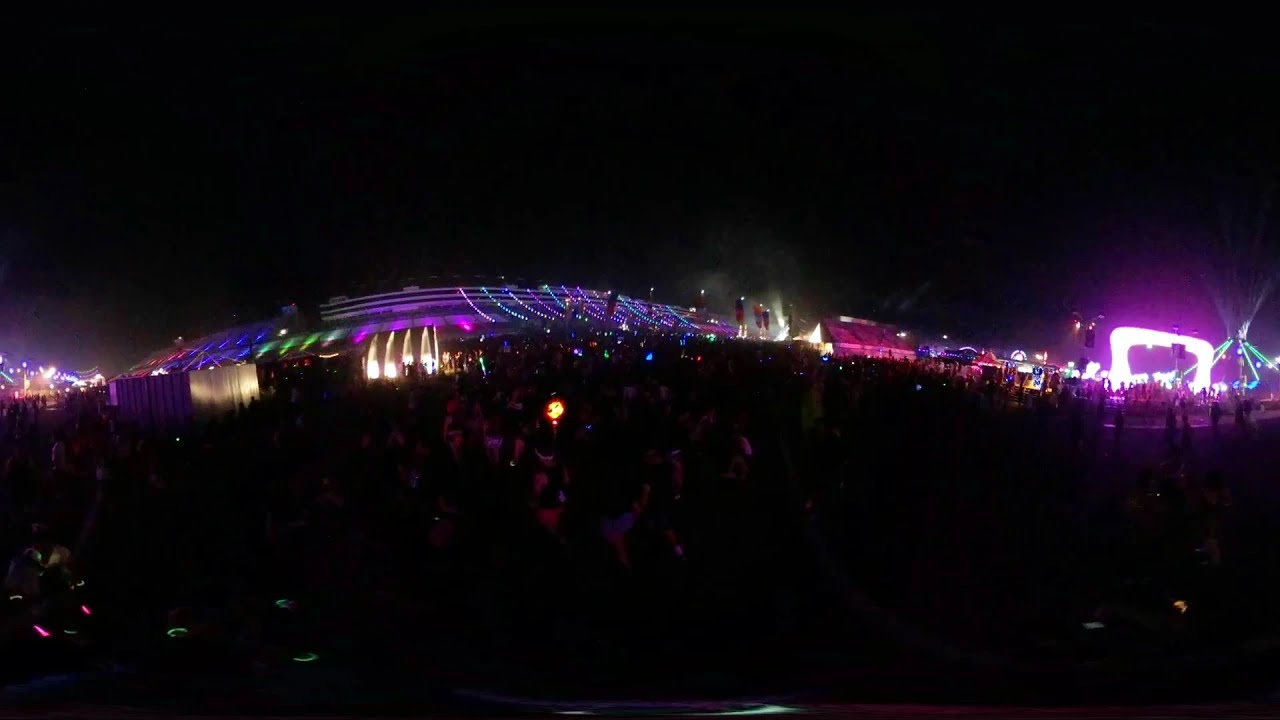This night-time photograph captures the vibrant, illuminated spectacle of an amusement park or festival. Dominating the right side of the image, a swing ride glows in blue, while behind it, a large white-lit frame or possibly an entryway adds a festive sparkle. In the middle of the image, a curved roof adorned with purple and green lights forms an arc-like structure, casting colorful reflections. Beneath this roof, strands of lights in purple, blue, white, and green drape elegantly. Scattered throughout the scene are small crowds of people, visible primarily as outlines against the bright, multicolored backdrop, giving a sense of bustling activity. The left side of the image features additional lights, including a green slash near the bottom, all set against the backdrop of a dark night sky. Various neon signs and backlit buildings line the background, contributing to the lively, nocturnal atmosphere.